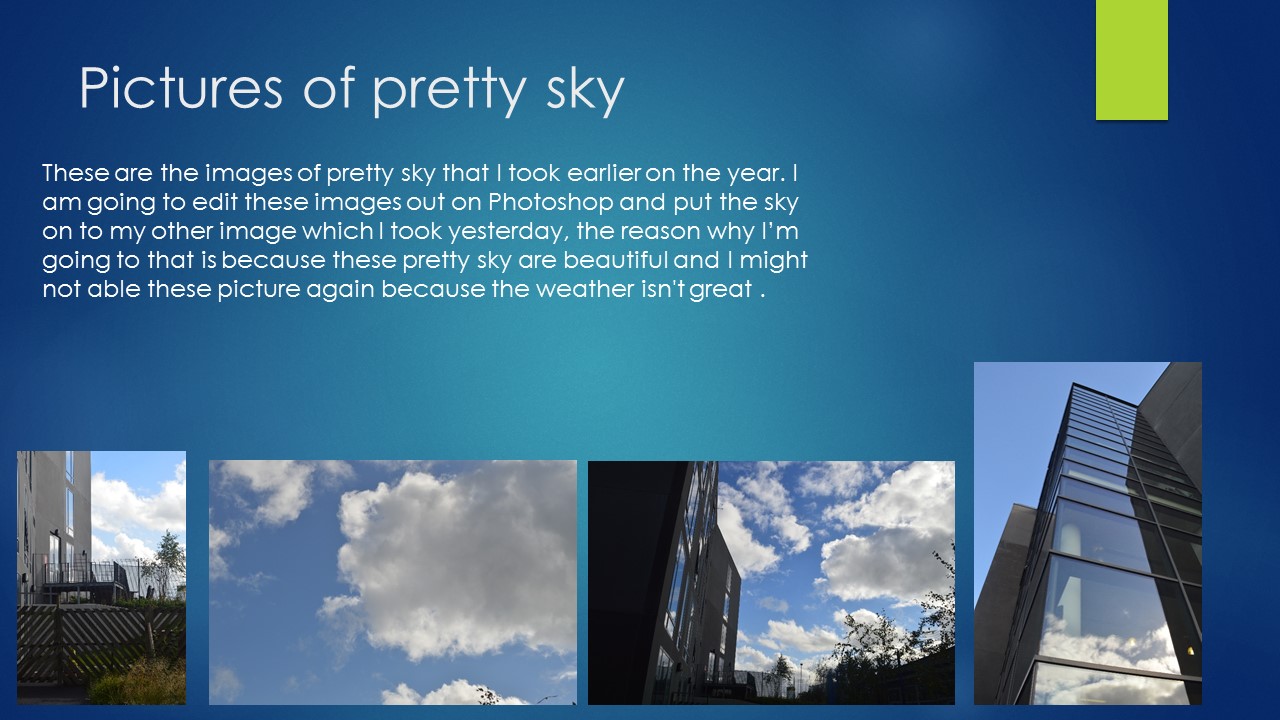An image features a PowerPoint slide with a blue background and white text. The top title reads "Pictures of Pretty Sky." Beneath the title, a block of smaller text states: "These are the images of pretty sky that I took earlier in the year. I am going to edit these images out on Photoshop and put the sky onto my other image, which I took yesterday. The reason why I'm going to do that is because these pretty sky are beautiful, and I might not be able to capture these pictures again because the weather isn't great."

At the bottom of the slide, four photographs are displayed from left to right. The first photo shows a fence in someone's backyard with the sky above it. The second photo features a blue sky with clouds. The third image captures a scene with trees and a building under the sky. The fourth and final photo presents a building with clouds reflecting off its surface. The images collectively depict various outdoor views, all highlighting different aspects of the sky. Additionally, there is a green rectangular area intruding from the upper right corner of the slide.